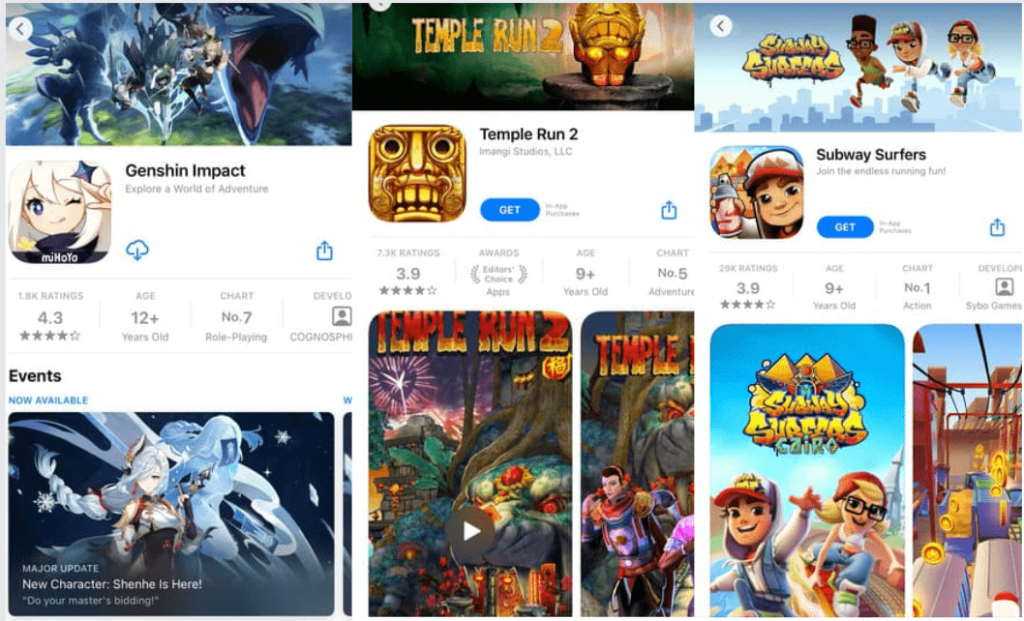The image showcases three app store screenshots of different popular mobile games side by side. 

- On the left is the app store page for Genshin Impact. The app has already been downloaded by the user, as indicated by the cloud icon with a down arrow. The profile picture for Genshin Impact features a character giving a salute, and the app boasts a rating of 4.3 stars. This game is suitable for players aged 12 and above. Below the profile picture, there are several in-game screenshots showcasing the game's features.

- In the middle, the app store page for Temple Run 2 is displayed. The profile picture is dominated by the iconic totem pole face, and the app has a rating of 3.9 stars. Temple Run 2 is recommended for users aged 9 and above. Like the Genshin Impact page, this screenshot also includes a series of images from the game under its profile section.

- On the right, the app store page for Subway Surfers is shown. The profile picture showcases the character holding a spray can, with a background depicting three characters running through a cityscape. The app holds a 3.9-star rating and is also recommended for users aged 9 and above. The bottom part of the page displays screenshots from the Subway Surfers game.

Each of these app store pages includes a white circle with a grey, left-facing arrow in the top left corner for navigation purposes.